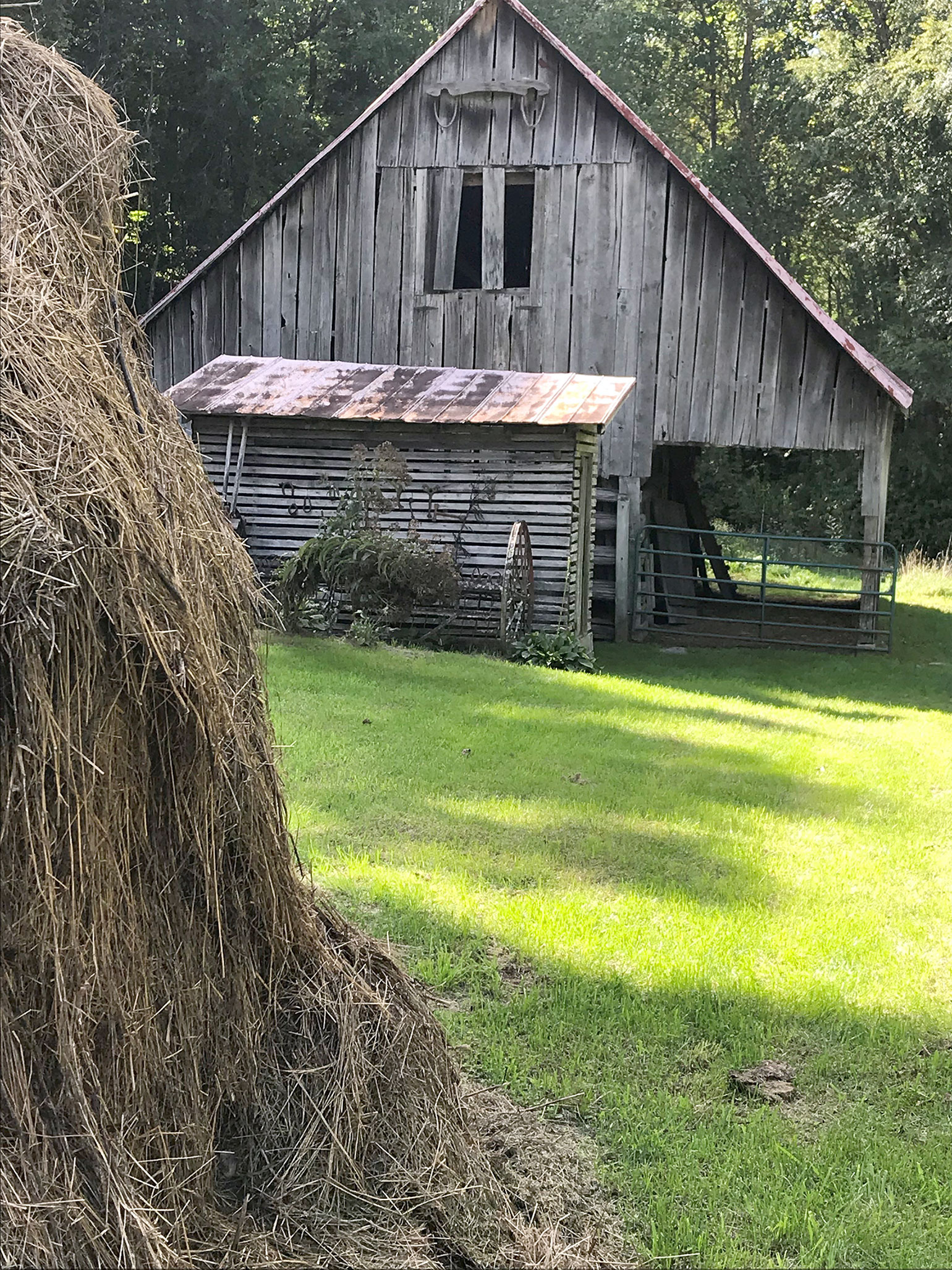This detailed color photograph captures an outdoor rustic scene dominated by a weathered barn with an angled V-shaped roof. Situated slightly in the background, the barn's wood appears aged and worn, hinting at years of exposure to the elements. In front of the barn, a partially visible metal shed with horizontal wood slats adds to the rural ambiance. The middle ground features a well-maintained, lush green lawn stretching across the scene, while the foreground on the left side boasts a large stack of hay, partially cropped and reaching from the bottom almost to the top of the photograph. Behind the barn, a dense forest bathed in sunlight casts dramatic shadows on the ground, highlighting the vibrant greenery of the day. The overall composition suggests a serene yet timeless countryside setting, with a blend of natural and man-made elements.